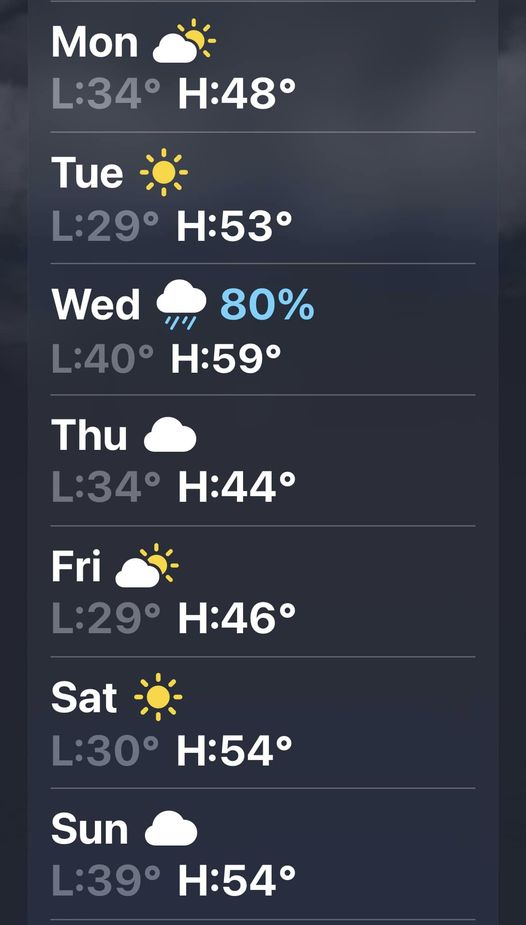This screenshot captures a detailed weekly weather forecast as displayed on a mobile weather app. The user interface features a sleek black background that contrasts sharply with the white text used to list the days of the week, from Monday through Sunday, in a vertical column. 

For each day, the forecast includes a weather icon positioned immediately next to the day's name, visually representing the expected conditions. The temperature details for each day are organized just below the icons, with the low temperature presented first and the high temperature following it. A thin line demarcates each day's forecast from the next, ensuring clarity and ease of reading.

The forecast details are as follows:
- **Monday**: Partly sunny icon. Low temperature: 34°F, high temperature: 48°F.
- **Tuesday**: Sunny icon. Low temperature: 29°F, high temperature: 53°F.
- **Wednesday**: 80% chance of rain (with the 80% highlighted in blue). Low temperature: 40°F, high temperature: 59°F.
- **Thursday**: Cloudy icon. Low temperature: 34°F, high temperature: 44°F.
- **Friday**: Partly sunny icon. Low temperature: 29°F, high temperature: 46°F.
- **Saturday**: Sunny icon. Low temperature: 30°F, high temperature: 54°F.
- **Sunday**: Cloudy icon. Low temperature: 39°F, high temperature: 54°F.

This well-organized forecast ensures that users can easily plan their week based on the anticipated weather conditions.